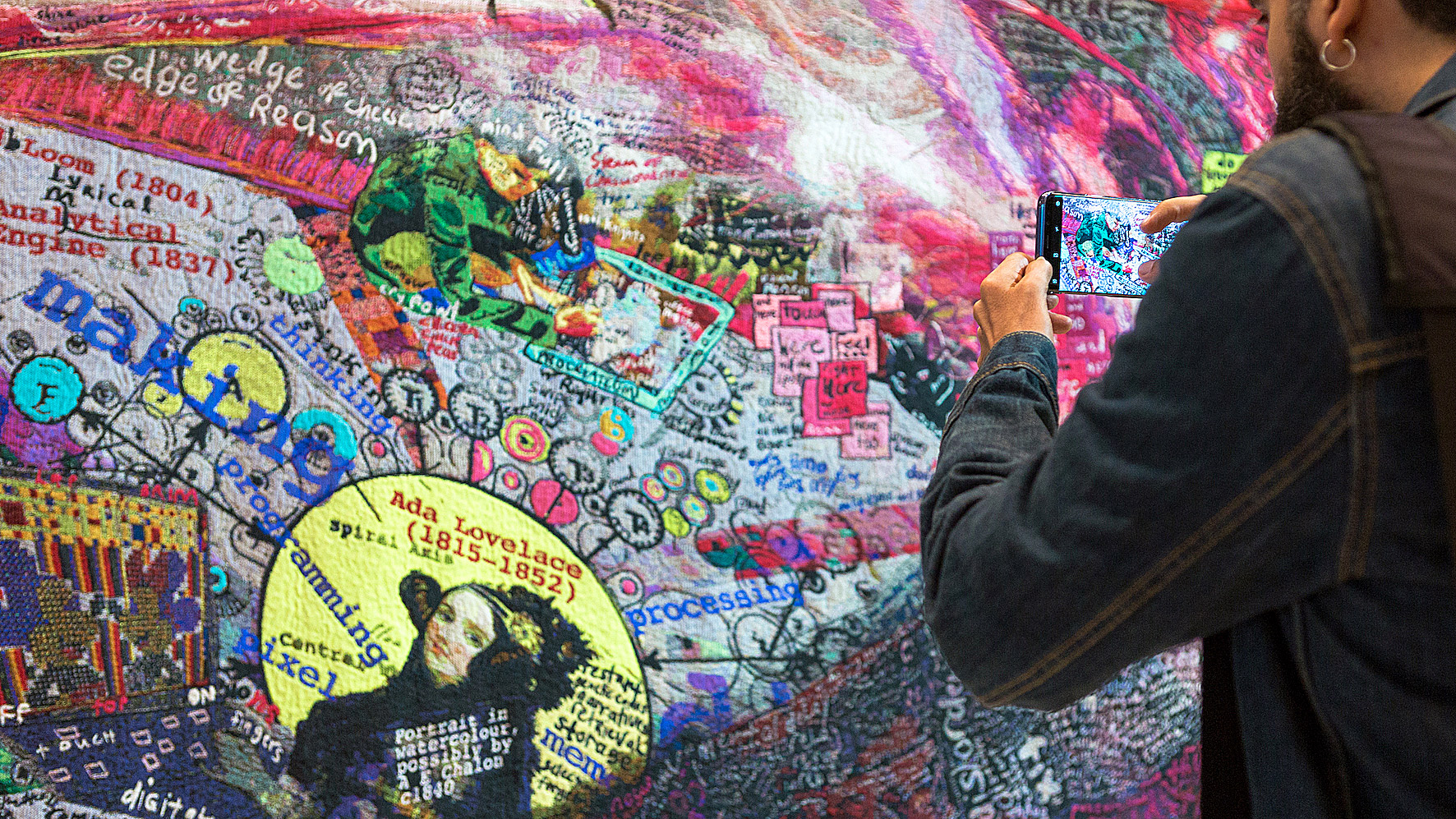In this vibrant outdoor photograph, a man in a dark blue denim jacket with tan stitching is captured taking a picture using his black smartphone. He stands on the right side of the image with his left arm extended, positioning the phone towards a vividly multicolored mural, which is seen on the screen of his device. This mural is a rich tapestry of colors, writing, and symbolic elements, prominently featuring a yellow circle at the bottom left containing a portrait of Ada Lovelace with the dates "1815 to 1852" in red text. Ada is illustrated with flowers and intricate details around her head, while additional text like "analytical engine (1837)" and "loom (1804)" mingles with colorful bubbles and shapes across the mural. The man, whose beard is flecked with gray and who sports a silver hoop earring in his left ear, also wears a brown shoulder strap or backpack. His phone captures the essence of the mural, creating a layered visual narrative as he photographs the detailed artwork just as he is being photographed himself. The mural teems with historical references and modern typography, blending vibrant blues, pinks, yellows, and a spectrum of other vivid hues to create a lively and intricate scene.